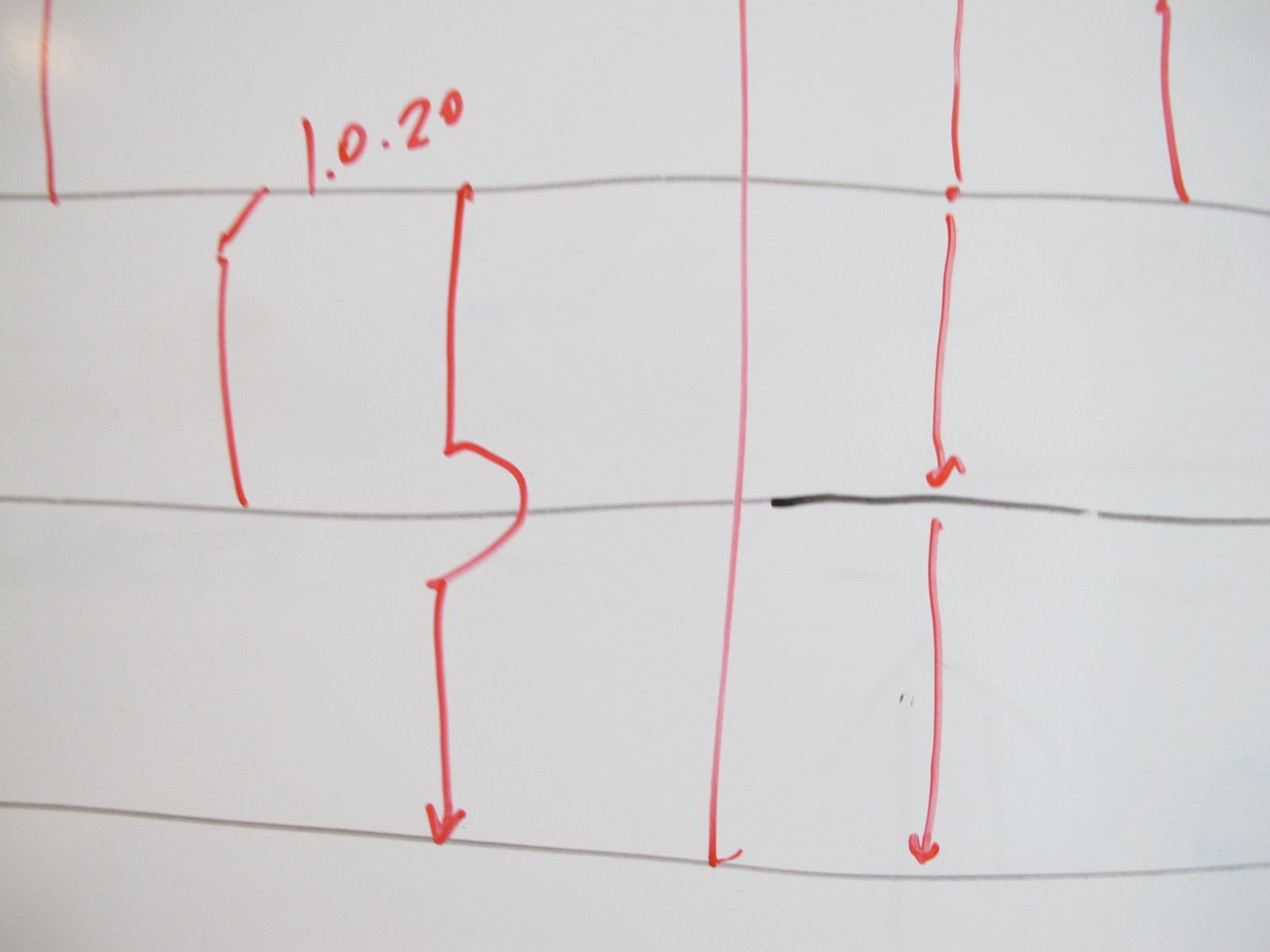This photograph captures a drawing on a white dry erase board, created using dry erase markers. The backdrop is entirely white, typical of such boards. At the top of the image, a small element vaguely resembling a camera flash is depicted. The main composition features a trio of fine grayish-black lines, with one appearing slightly faint as if the marker was running low on ink. Overlaying these are multiple red line markings, some of which culminate in downward-pointing arrows. Among these red lines is a distinctive marking with a circular shape at its center. Additionally, inscribed in red near one of these lines is the notation "1.0.20". The drawing contains no other objects, ensuring that the viewer's focus remains on the detailed interplay of gray and red markings against the pristine white background.